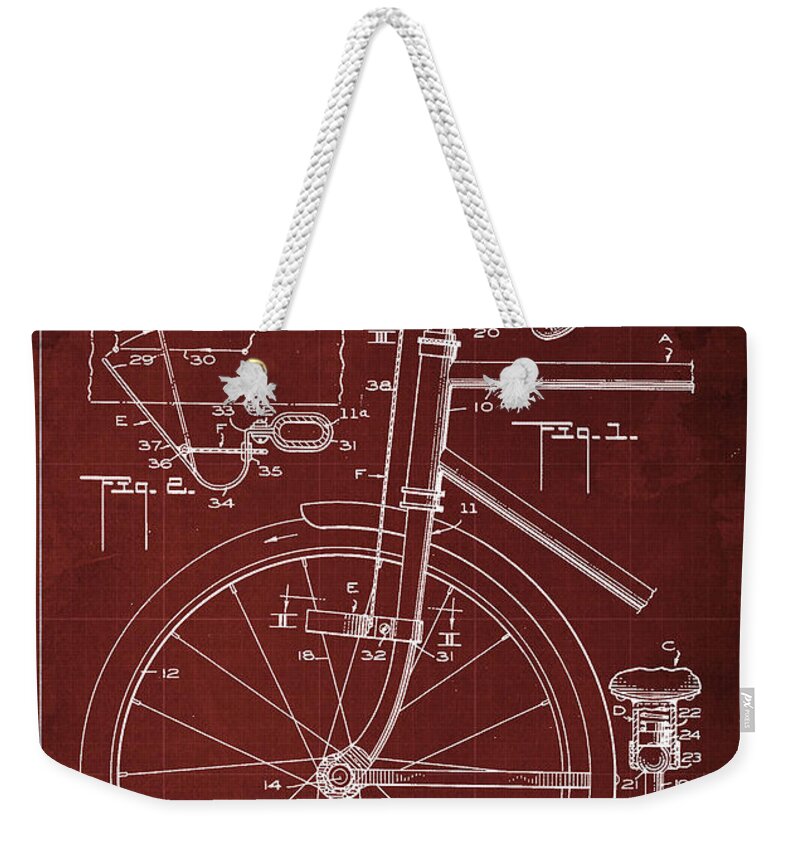The image showcases a large canvas tote bag with white rope handles that resemble shoelaces. The fabric of the bag is a deep burgundy, maroon color with faint, scattered red lines in the background. The central graphic on the bag is a detailed, white schematic drawing of a bicycle. This diagram features a zoomed-in section of a bicycle wheel, complete with spokes, a mud guard, and the forks. The bicycle schematic also includes outlines of a long rifle and various mysterious letters pointing to different elements of the drawing. At the bottom left corner, there's an additional small, indistinct object connected to the bicycle. The overall design appears technical and complex, resembling an instructional figure with a title "figure one," and gives the impression of illustrating how to assemble a bicycle.